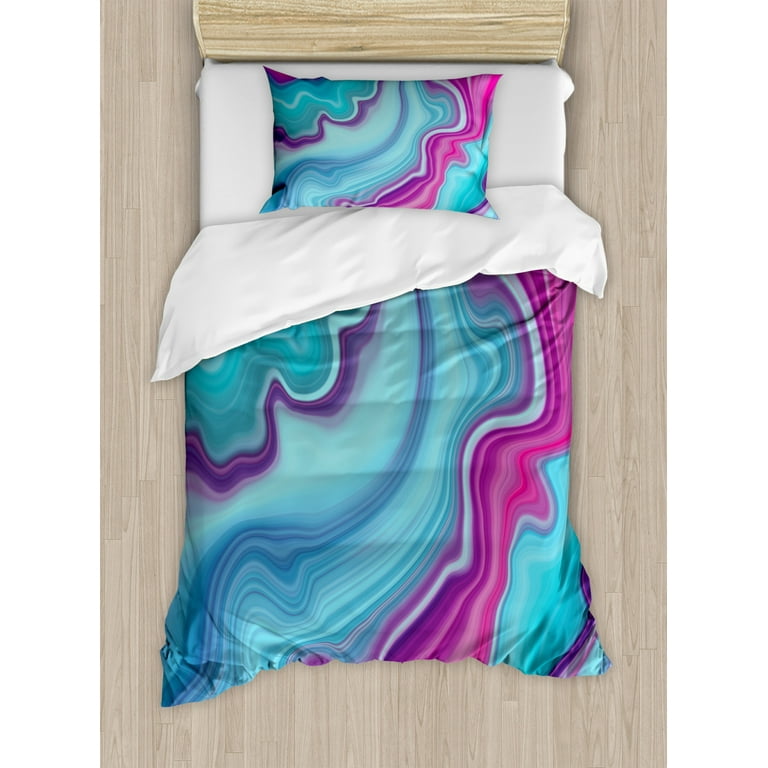This image is an aerial view of a bedding mock-up, showcasing a bed positioned on a grayish wooden floor. The bed features a white fitted sheet, with the comforter pulled down to reveal the underside. The comforter and the single pillow share an identical, eye-catching design. This design consists of swirling patterns in shades of blue, turquoise, teal, pink, and purple, reminiscent of oil on water or paint spreading across a canvas. The headboard is wooden, providing a stark yet complementary backdrop to the vibrant, almost cotton-candy-like colors of the bedding. This visually compelling composition, likely concept art, emphasizes the unique and artistic design of the comforter and pillow.